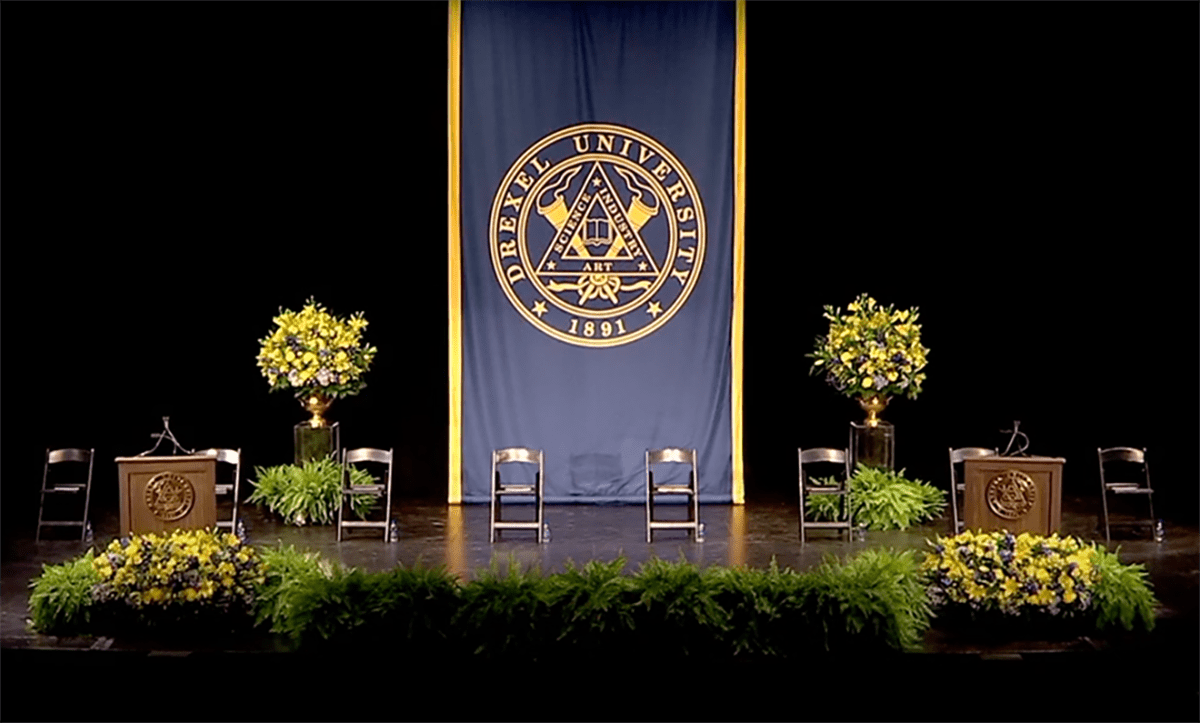The photograph captures an indoor stage set against a black background, exuding an educational ambiance. Centered on the stage is a dark blue curtain adorned with an emblem featuring a triangular shape flanked by two torches. The circular text reads "Drexel University 1891," with additional text inside the triangle stating "science and industry" along with a book in the center. A harmonious arrangement of silver chairs lines the stage, accompanied by two brown wooden podiums, each equipped with a microphone. On either side of the curtain, potted plants complement the setup, while vases atop pedestals burst with vibrant yellow flowers. At the base of the stage, a lush array of green grass, sea ferns, and blue and yellow flowers adds a touch of nature, creating a vivid and inviting scene.